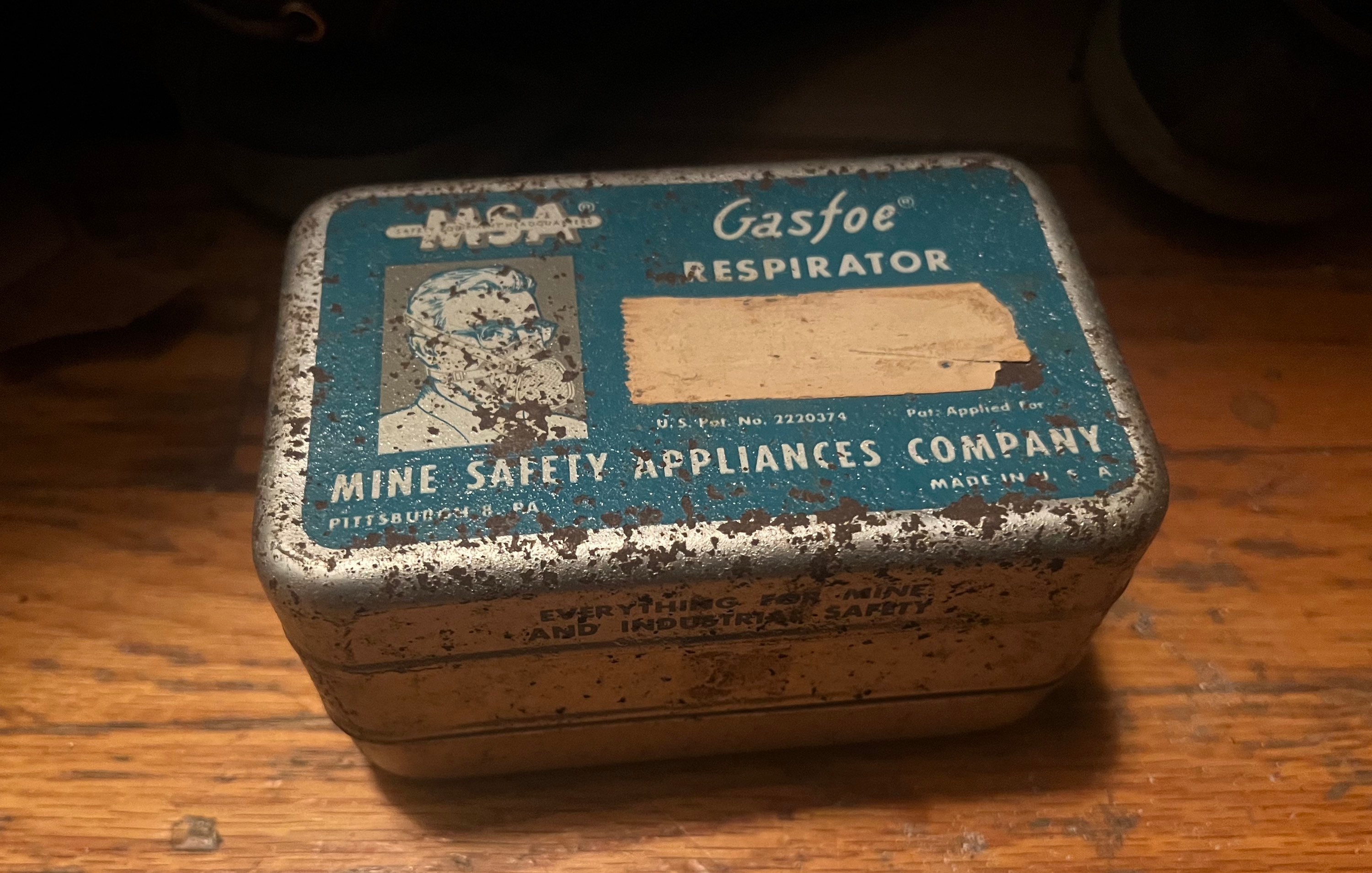This image depicts an extremely old, rectangular-shaped metal tin can with rounded edges, sitting on a brown wooden surface. The tin is predominantly silver, heavily speckled with rust spots, and has a blue top. The top is adorned with various texts and illustrations. In the upper left-hand corner, "MSA" is written in white text. Centered on the lid, it says "Gas Pho Respirator." To the left, beneath the letters "MSA," there is a blue and white illustration of a man with a beard and glasses, wearing attire suggesting he is a doctor. Adjacent to the man's image is a piece of yellowed tape, likely covering some information. Below the illustration, it reads "Mine Safety Appliances Company." Additional details include "USPAT number 2220374, PAT applied for." Around the side of the lid, in black uppercase letters, it says "EVERYTHING FOR MINE AND INDUSTRIAL SAFETY," emphasizing the vintage and industrial nature of the tin.